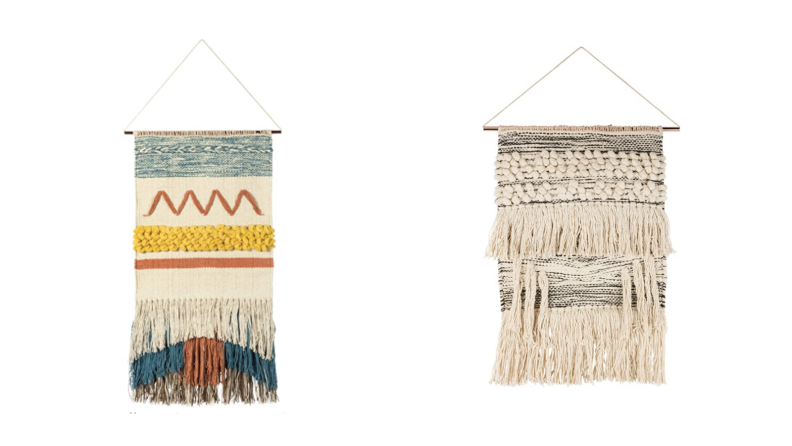This image features two intricately crafted decorative pieces, both suspended from a triangular wooden hanger. The piece on the left is vividly colorful, evoking elements of Indian culture. It showcases a thick blue stripe at the top followed by red squiggly patterns reminiscent of mountains or waves. Below this lies a yellow segment that resembles grains or corn, accentuated with a thin red stripe. The main fabric transitions into a white section, culminating in loosely hanging threads of white, blue, and gray, with a red area embedded within the blue threads. The right decoration contrasts with a more subdued palette of grays and blacks but compensates with intricate fabric patterns. This piece features stripes at the top and multiple sets of tassels—one set hangs in the middle and another at the bottom, giving it a balanced yet elaborate appearance. Both pieces highlight the craftsmanship through their detailed designs and repeating tassels.